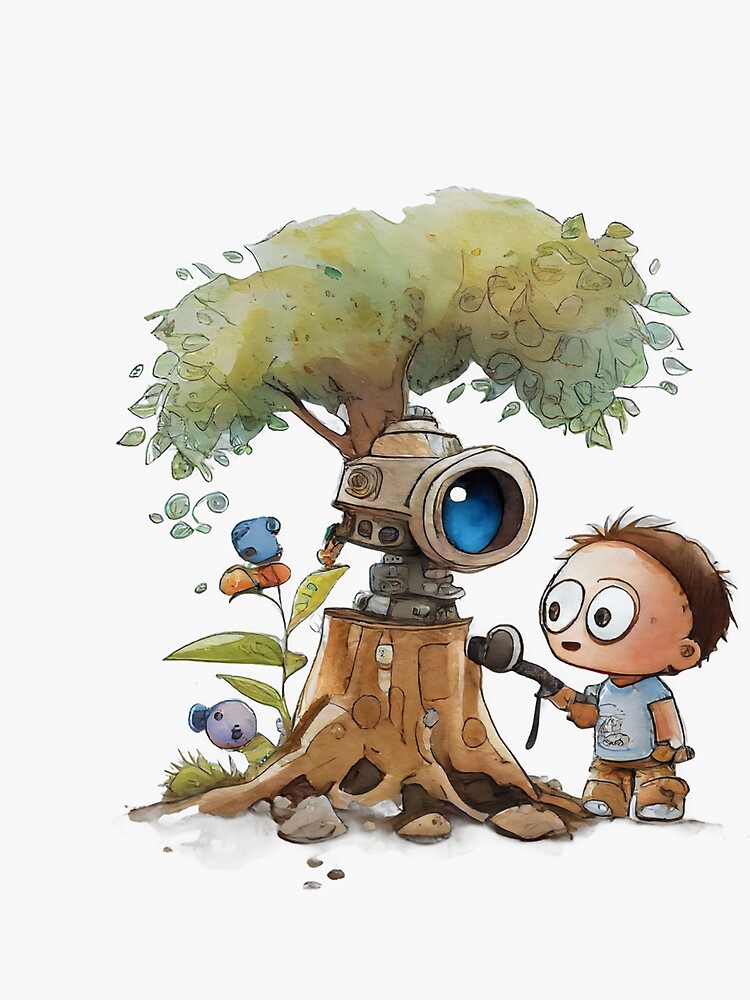The image is a cartoon-style drawing on a white background featuring a central tree stump, partially integrated with technology. The tree stump is predominantly brown except for the gray section where the technology is embedded. This section houses a large, blue fish-eye lens, slightly oriented towards the right. Emerging from the stump, the tree continues to grow with brown extensions and green leaves and shrubbery in a cartoonish style. 

To the right of the tree stands a cartoon-style boy with exaggeratedly large eyes, small pupils, and dark hair. He is dressed in a blue shirt with some kind of design, brown pants, and wears a watch. In his left hand, he holds a black tool, which he appears to be using on the technological part of the tree. 

To the left of the tree, a small green plant is growing, accompanied by green and blue cartoon shapes near its base. Additionally, there are orange and blue cartoon shapes at the top of the image. The scene suggests the boy might be interacting with the technology on the tree, possibly in preparation for filming something.